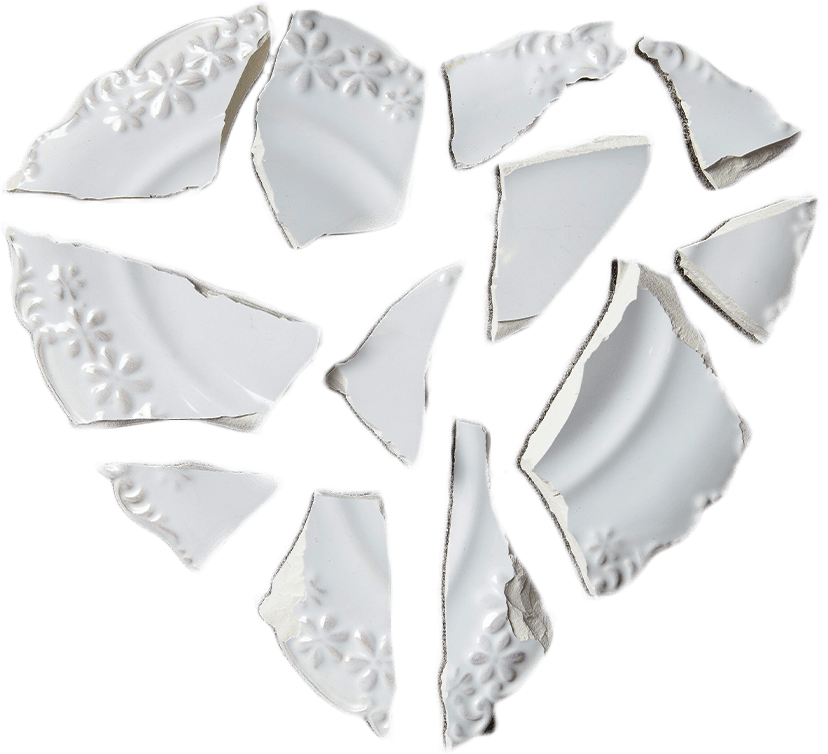This image depicts an aerial shot of broken white porcelain or ceramic shards arranged to form the outline of a heart against a stark white background. The fragments appear to be from a delicate plate or saucer, likely heart-shaped originally, as evidenced by the haphazard layout that suggests this form. Each piece is meticulously placed, revealing ragged, broken edges, and tiny embossed floral patterns, possibly daisies, that add intricate detailing. The stark simplicity of the white ceramic against the white background accentuates the delicate and fragile nature of the original plate, evoking a sense of nostalgia and loss, reminiscent of fine, delicate plates often treasured in the past.